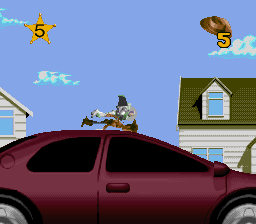In this digital depiction from a video game, a burgundy car with a sleek, sloped back is shown in motion, either heading left or right. Clinging to its roof is some sort of creature, though its details are unclear. The car is driving past two white houses; the house on the right has distinct gables and can be seen over the hood. Both houses have strikingly blue windows and greenish roofs. The right-side house possibly has a doorway, though it's not clearly visible. Additionally, there is an emblem resembling a star with the number five inside, as well as a hat that also features the number five, adding to the intrigue of the scene.